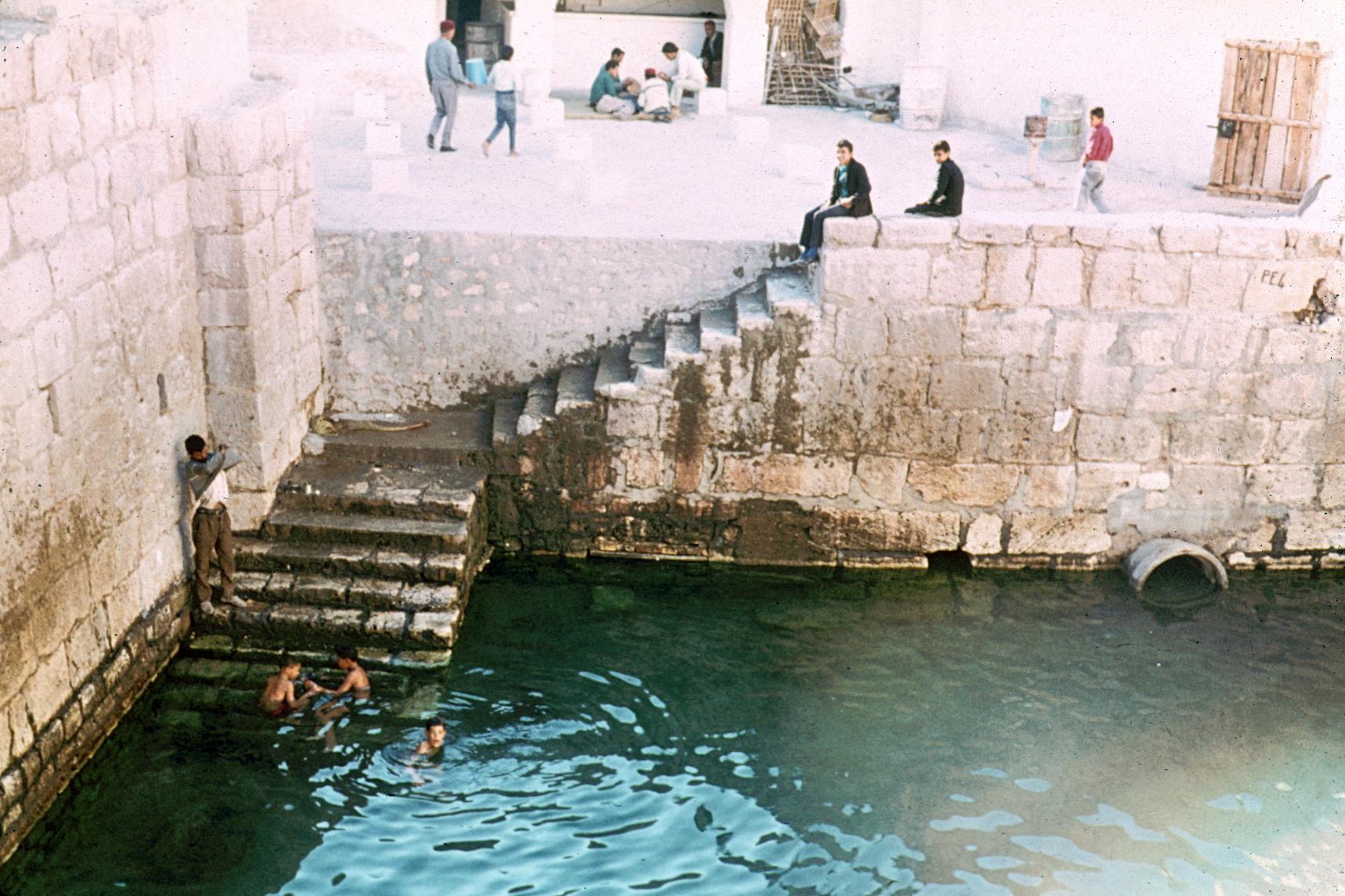The image depicts a bustling outdoor scene in a picturesque European locale, resembling a stone castle setting. This multifaceted composition showcases a pool of greenish-blue water at the bottom of two flights of wet stone and concrete stairs. To the right of the stairs, there is an old wooden door set into the masonry wall. Several people, including children swimming in the water and men in black attire sitting on the stairs, animate the scene. One man is captured mid-action, attempting to remove his shirt at the bottom of the stairs, likely preparing to swim. The stone walls and stairs, along with the pool, are surrounded by earthy tones of white, tan, and gray. At street level above, a man and a woman walk along the concrete path while others sit in a small enclave, observing the activity below. Adjacent to them, a group of four people can be seen sitting around what seems to be a table, engaging in conversation. A large culvert-like structure punctuates the middle of the wall, adding to the historical ambiance of the setting. The bright daylight underscores the lively atmosphere, with various groups of individuals scattered at different elevations, enjoying the vivid, communal space.